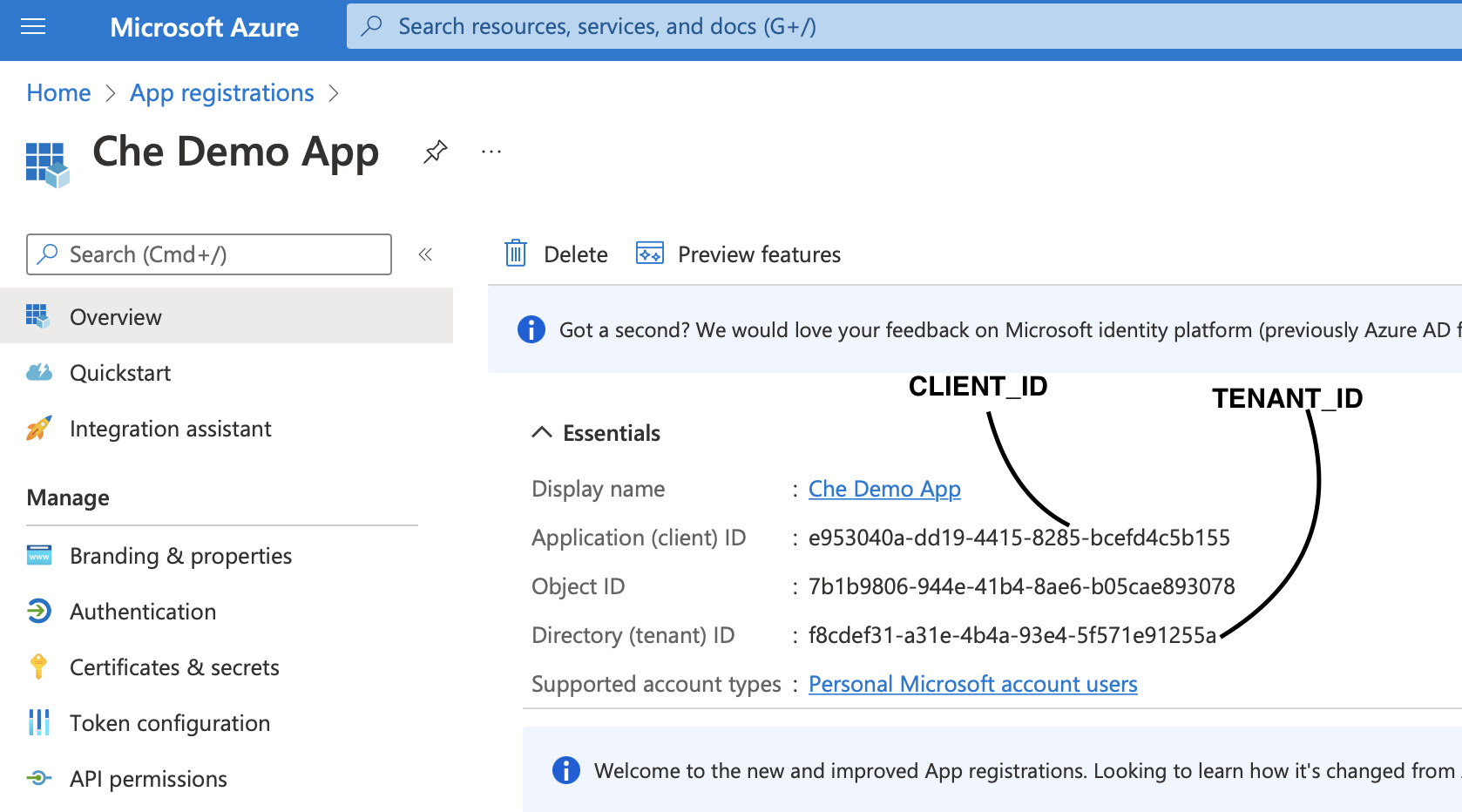The top part of the image displays a blue banner stretching across the width. On the left-hand side, there are three horizontal white lines, followed by the text "Microsoft Azure." Adjacent to this text is a light blue search box, truncated on the right side. Within this box, there's a blue magnifying glass icon, and the text reads "Search resources, services, and docs." In parentheses next to this, it says "(G + /)."

Beneath this, the background is white. A blue heading reads "Home > App registrations," followed by the black text "CHE Demo App." There is an outlined black search box that says "Search," complemented by the parentheses text "(CMD + /)."

Continuing below, the black text lists various sections: "Overview," "Quickstart," "Integration assistant," "Manage," "Branding and properties," "Authentication," "Certificates & secrets," "Token configuration," and "API permissions." On the right-hand side, a blue trash can icon is labeled "Delete" in black text. Below it, the text "Preview features" appears in black.

A blue border runs across, containing a blue circle with a white "i" icon inside. Next to this is the black text: "Got a second? We would love your feedback on Microsoft identity platform (previously Azure AD)." The text cuts off after this point.

At the bottom, a blue border reads, "Welcome to the new and improved App registrations. Looking to learn how it's changed from," but the sentence is cut off and cannot be fully read. In between these sections, additional black text details key application information: "Essentials," including "Display name," "Application (client) ID," "Object ID," "Directory (tenant) ID," and "Supported account types."